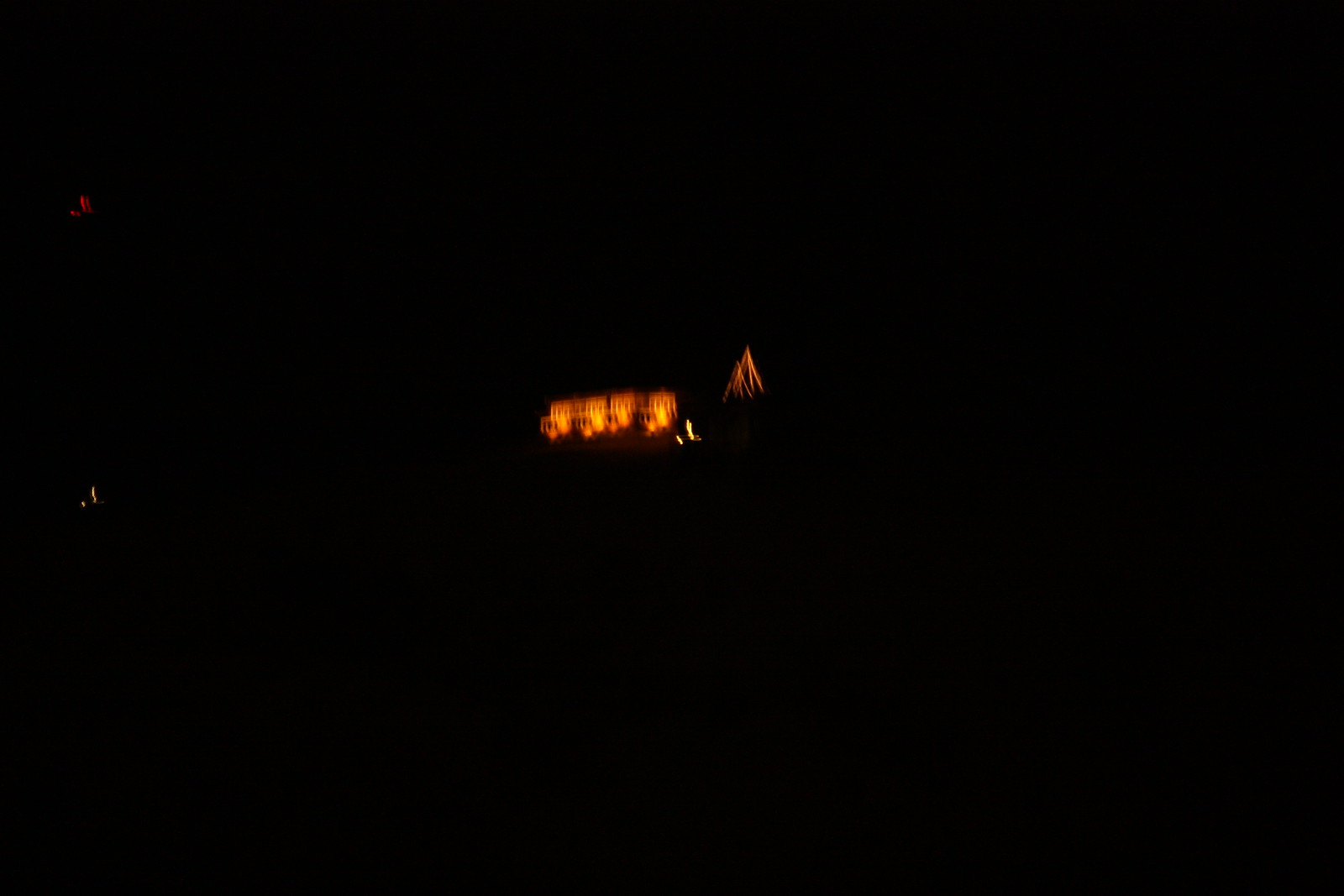In this very blurry nighttime photograph, the entire frame is enveloped in near-total blackness except for a few pinpoints of light and a central glowing structure. The center of the image features an orange-lit structure, likely a house or a garage, adorned with four large, bright orange lights. Surrounding the main structure, there are various smaller lights: a small red light in the top left corner, a small yellow light in the middle left, and a couple of yellow light rectangles along with orange lit-up triangles at the bottom right. Additionally, there are some subtle orange and amber reflections scattered around. Despite the overall darkness and indistinct details, the illuminated elements create a focal point that highlights the festive atmosphere, reminiscent of Christmas decorations.